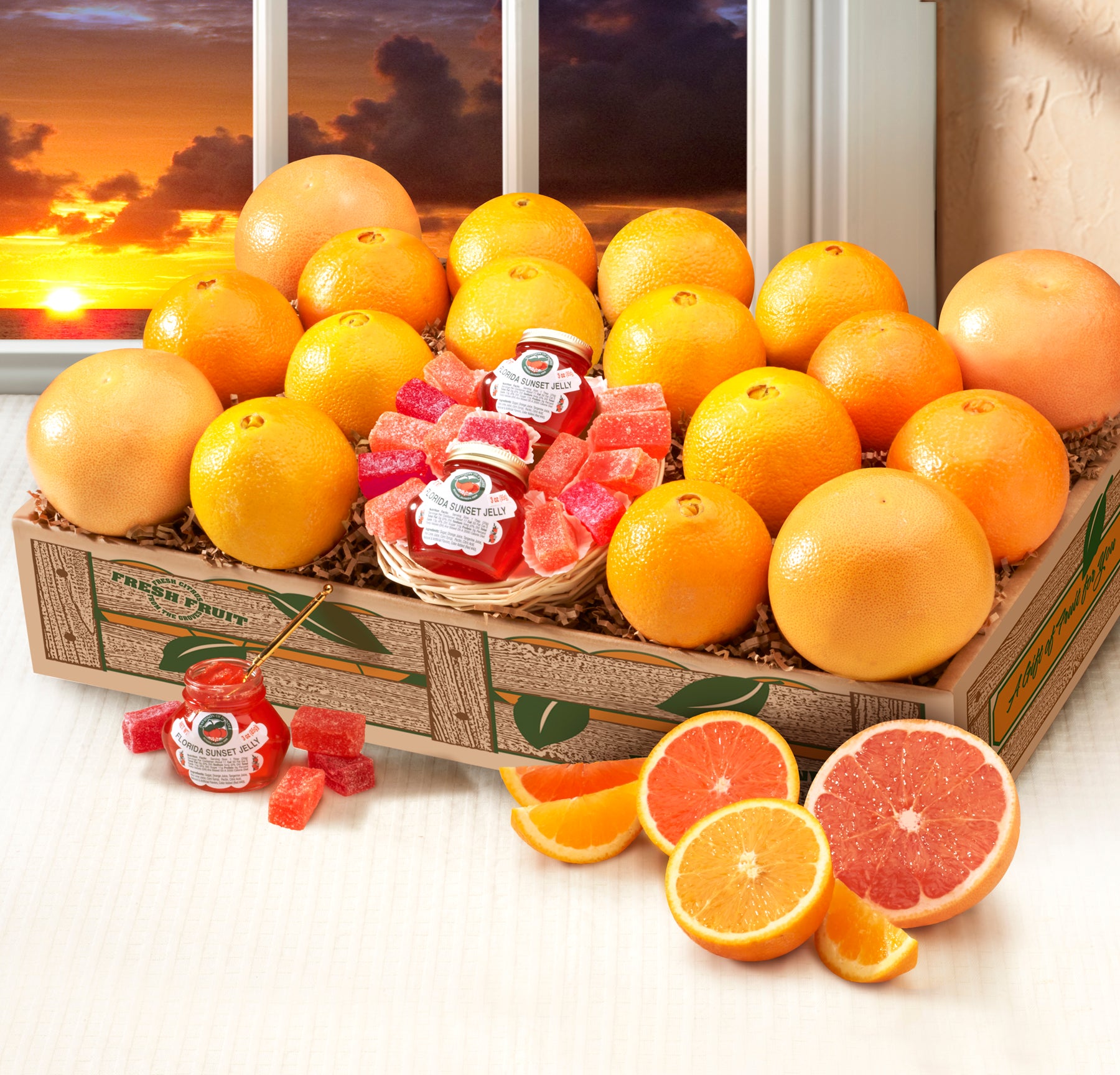This marketing photo showcases an exquisitely arranged crate of fresh citrus fruits and artisanal products. The wooden box, padded for effect, is filled with a vibrant assortment of oranges, grapefruits, and possibly blood oranges, all shining and meticulously positioned. At the center of this colorful medley sits a charmingly displayed basket containing jars of preserves and neatly cut blocks of sugared candies, suggested to be crafted from these citrus fruits. In front of the box, on a plain matte white counter, some oranges are artistically cut open, revealing their juicy interior, with various wedges scattered around. An open jar of preserves with a spoon in it, along with some of the candied products, add to the enticing display. The background features a large window framed in white, through which a stunning sunset over a cloudy sky adds a warm, serene glow, painting an idyllic ambiance that enhances the attractiveness of these citrus delights. The scene, although possibly edited, beautifully blends elements to create a visually appealing portrait of fresh fruit and gourmet treats.